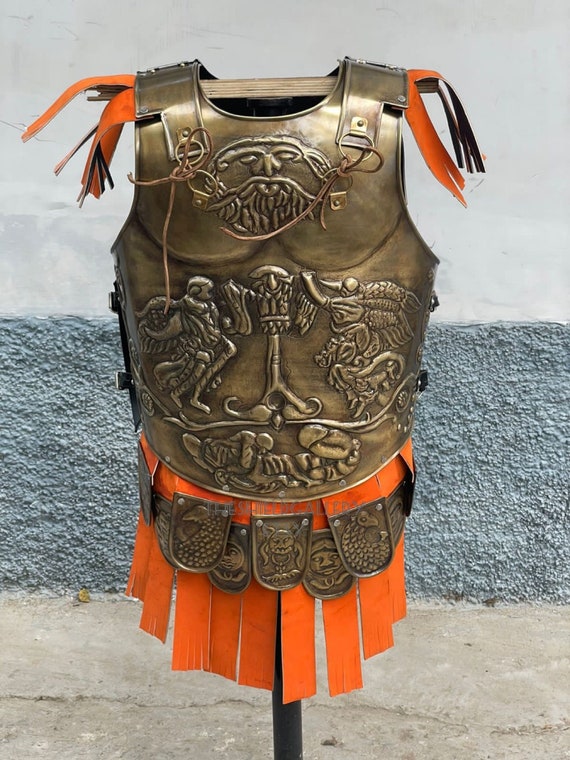This is an image of a bronze-colored metal breastplate on display, possibly outdoors, against a rough rock backdrop. The breastplate, intricately embossed with an image of two knights flanking a statue and a stylized animal resembling an alligator, is hanging on a wooden hanger mounted on a stick-like structure. Orange fabric strips, frayed at the ends, drape from the shoulders and form a skirt below the breastplate, evoking the appearance of a grass skirt. Additionally, a belt composed of curved metal segments, each adorned with various embossed figures—including faces and fish—encircles the waist area. These elements suggest historical armor, reminiscent of what might have been worn by a Renaissance-era military figure. The entire setup is likely in a museum or similar exhibition space.